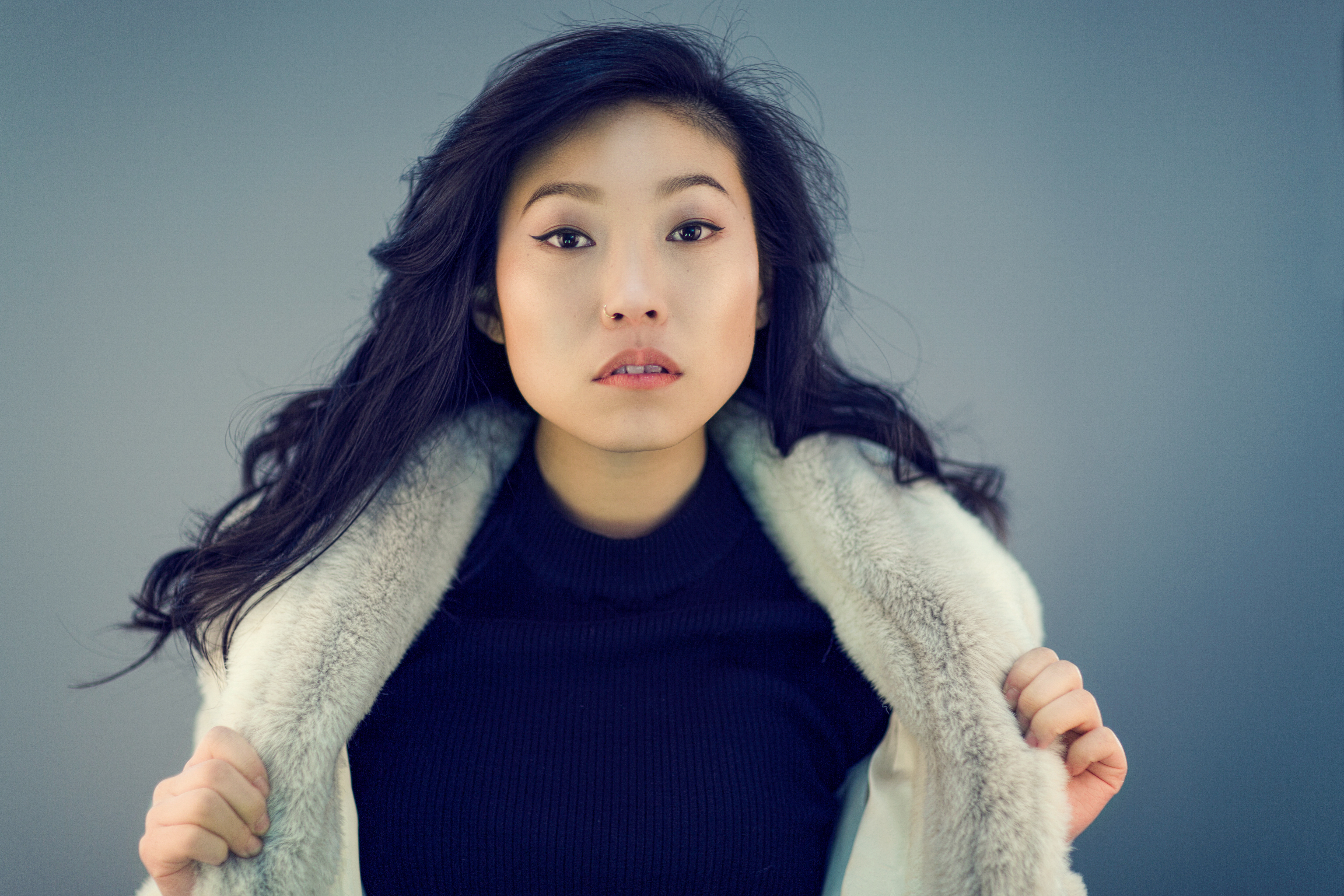This is a horizontally aligned rectangular photograph of an Asian woman with long, slightly wavy black hair extending past her shoulders. She has tan skin and is wearing subtle cat wing eyeliner, giving her a serious expression with slightly parted lips that reveal her front teeth. The image captures her in a pale, possibly faux fur coat that she holds slightly open with her left hand, which appears to have a ring on it. Underneath the coat, she is dressed in a dark-colored, possibly black, high-necked t-shirt. The backdrop is a gradient light blue that becomes lighter near the woman, suggesting that a light is shining on her. The photograph exudes a modern style, likely captured within the last 20 to 30 years.